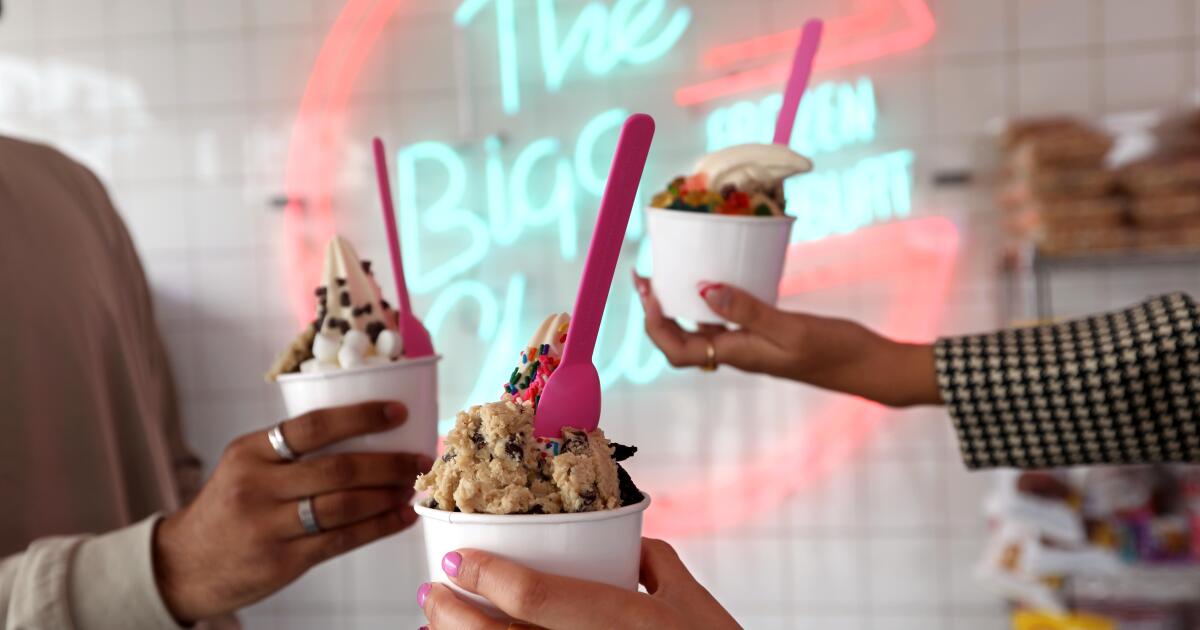The image captures the vibrant interior of a frozen yogurt shop. In the foreground, three distinct hands are prominently holding white disposable cups brimming with frozen yogurt, each adorned with unique toppings. On the left, a hand with dark skin, wearing two silver rings, holds a cup topped with a peak of yogurt embellished with chocolate chips and miniature marshmallows. At the center, another hand presents a cup featuring frozen vanilla yogurt garnished with colored sprinkles and chunks of chocolate chip cookie dough. To the right, a hand in a black and white houndstooth checked sleeve holds a cup topped with multicolored gummy bears. Every cup has a bright pink plastic spoon sticking out.

In the background, the shop’s ambiance is highlighted by a neon sign on a white tiled wall, featuring an orange neon circle with partially legible turquoise text, presumably spelling out "Frozen Yogurt" along with some additional unreadable characters. Industrial shelving stocked with supplies is faintly visible, adding to the professional yet lively atmosphere. The combination of bright colors, varied yogurt toppings, and personalized details paints a vivid scene of a bustling yogurt shop experience.